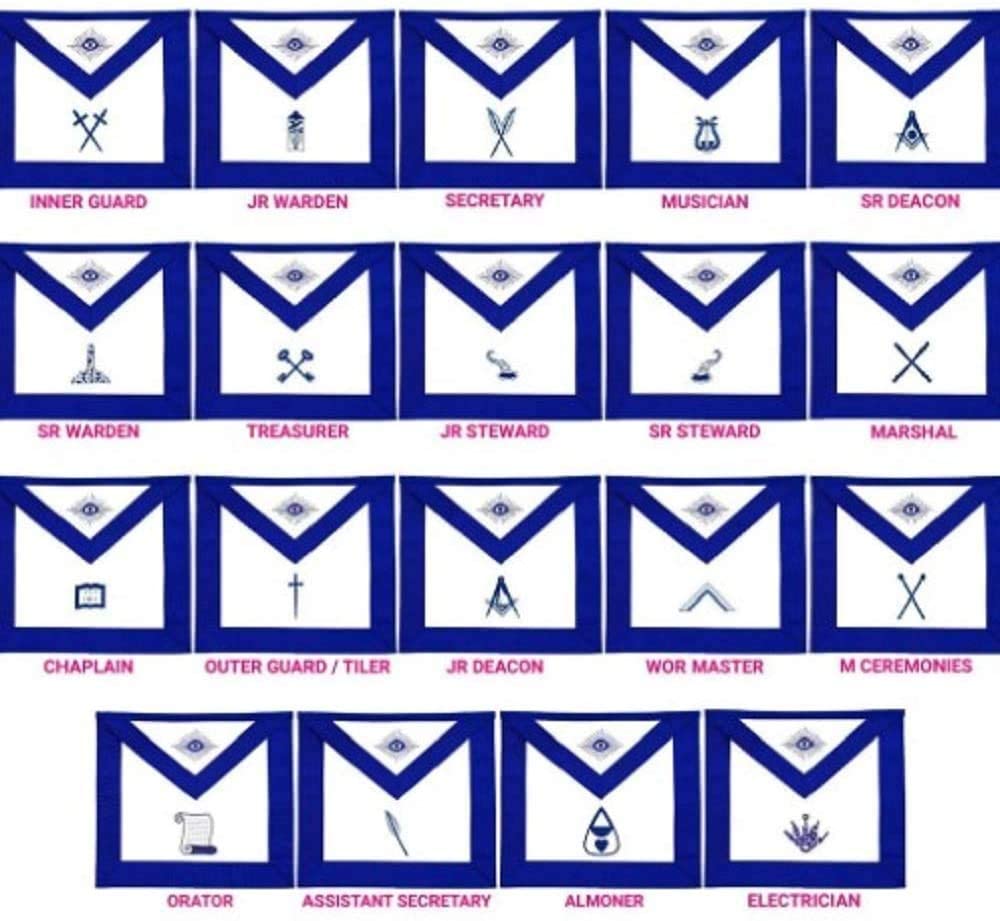The image depicts a chart with a white background, featuring 20 blue-and-white envelope-like icons arranged in four rows. Each envelope has a distinct symbol on its flap and a corresponding label beneath it in capital pink letters. The first three rows each contain five envelopes, while the fourth row has four. The icons symbolize different positions or roles, with examples such as a harp for musician, crossed quills for secretary, crossed swords for inner guard, and a sword for outer guard. The labels provide descriptions like "In Regard," "J.R. Warden," "Secretary," "Museum," "Senior Deacon," and additional roles such as "Senior Warden," "Treasurer," "Junior Steward," "Senior Steward," "Marshal," "Chaplain," "Outer Guard/Tiller," "Junior Deacon," "War Master," "Master of Ceremonies," "Orator," "Assistant Secretary," "Almoner," and "Electrician." Each position is represented with a unique symbol, offering a comprehensive and organized display of various roles.